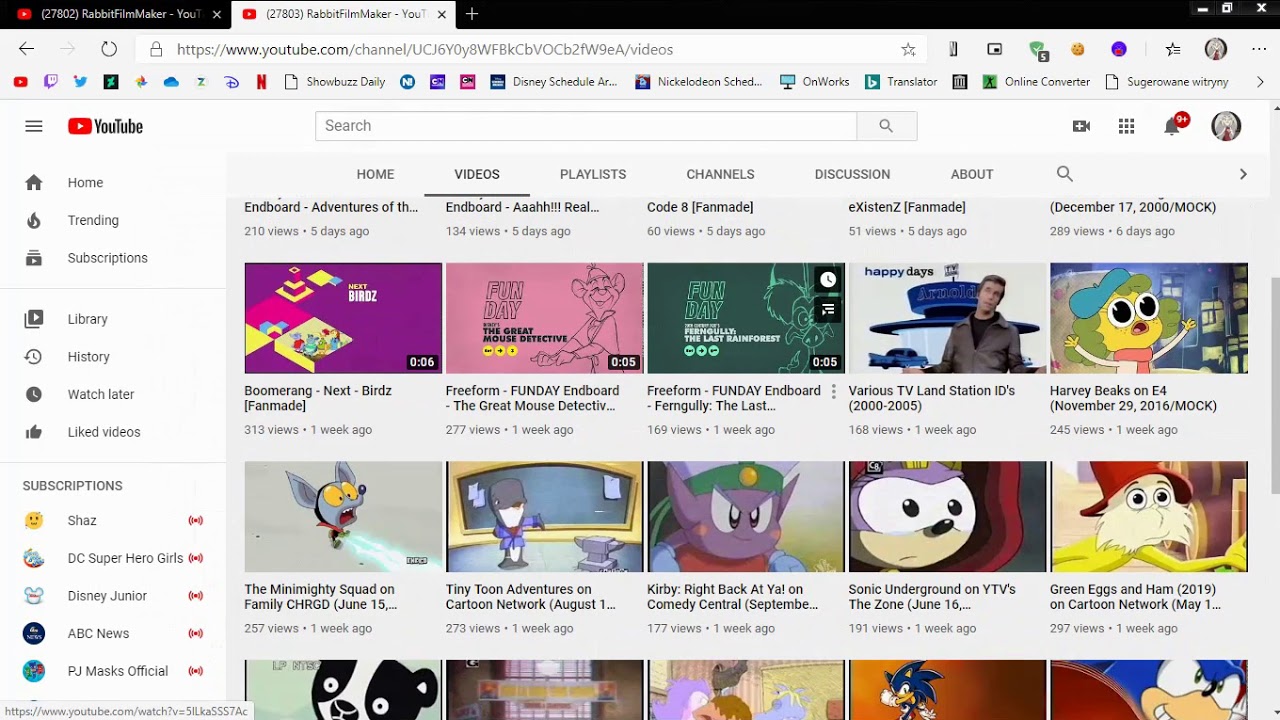The image is a rectangular screenshot with its longer sides extending horizontally. It appears to capture a YouTube interface displaying 12 video thumbnails in a grid layout. Each thumbnail features cartoon-style graphics and displays content from various animated series. The titles include "Boomerang Mix Binds," "Mini Mighty Squad Family Charge," "Tiny Toon Adventures," "Kirby: Right Back at Ya! Comedy Central," "Sonic Underground on YTV," "Green Eggs and Ham on Cartoon Network," and a few others.

On the left side of the interface, there is a vertical navigation column listing options such as "Home," "Trending," "Subscriptions," "Library," "History," "Watch Later," and "Liked Videos." Further down, under the "Subscriptions" section, channels like "Shaz," "DC Superhero Girls," "Disney Junior," "ABC News," and "PJ Masks Official" are listed.

Above the video thumbnails, there are several tabs labeled "Home," "Videos," "Playlists," "Channels," "Discussion," and "About," with the "Videos" tab currently selected. The entire layout mimics the classic YouTube homepage, emphasizing user subscriptions and recommended animated content.